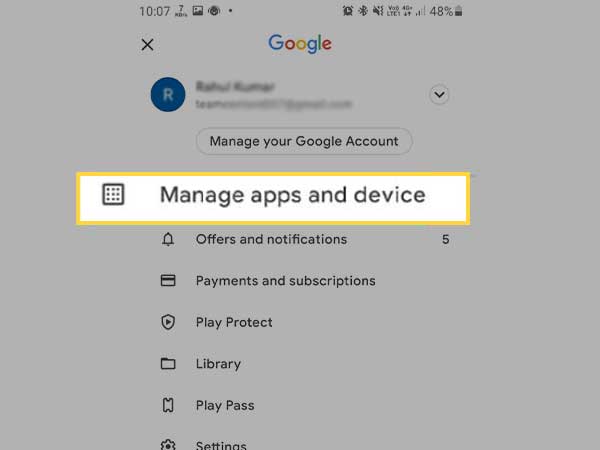This image is a square-cropped screenshot of the Google interface, specifically featuring the top section of the Google homepage or a Google search page. Dominating the top center is the iconic "Google" logo. To the left of the logo, there is an "X" symbol for closing the overlay. Below this, a user account section is visible. On the left side of the account section is a blue circular default profile picture featuring a capital letter "R" in the center. To the right of this default profile picture, the user's account name and email address are displayed, though they are pixelated for privacy. Further to the right, there is a drop-down arrow indicating additional options. Beneath the account name and email address, a prominent "Manage your Google Account" link is displayed.

Directly below this link, the first category listed is "Manage apps and device." This specific category has been edited for emphasis: it is enlarged and enclosed within a yellow box, and this highlighted version is pasted back over its original position to make it appear zoomed in. Following this highlighted category, six more categories are listed in smaller text, namely "Offers and notifications," "Payments and subscriptions," "Play Protect," "Library," "Play Pass," and "Settings."